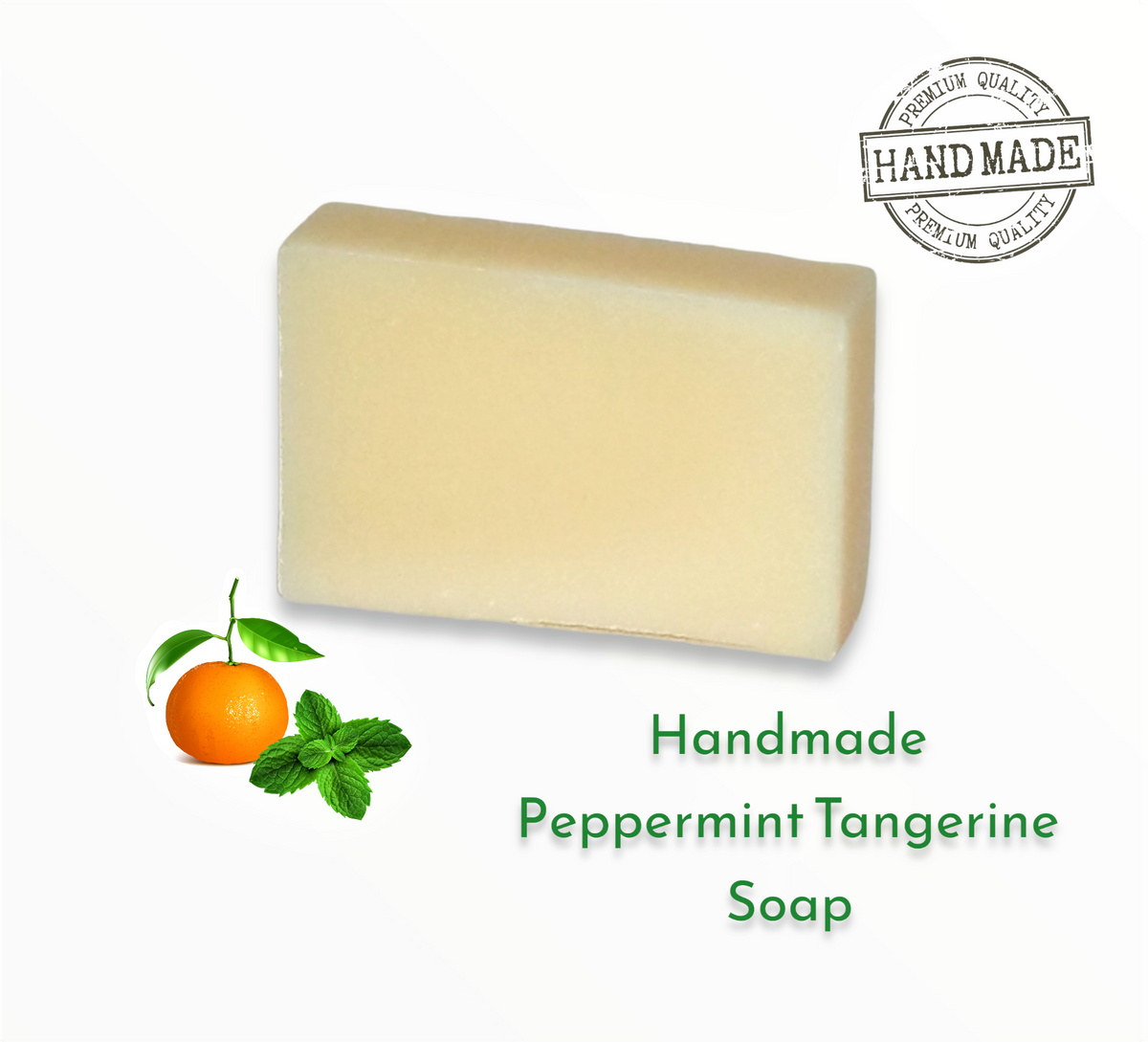The image is an advertisement for a tan, creamy beige colored soap block that is almost perfectly centered against a white background. Below the soap, green text with a hazy drop shadow for visibility reads "handmade peppermint tangerine soap." To the lower left of the soap, there is a detailed illustration of a tangerine standing upright with a small stem and leaves, accompanied by a peppermint plant featuring four prominent leaves. In the top right corner of the image, a circular seal of quality is displayed, with the words "premium quality" inscribed around its upper and lower parts, and the word "handmade" crossing through the middle of the circle in a rectangular banner. The imagery and text collectively emphasize the high-quality, handmade nature of this peppermint tangerine soap.